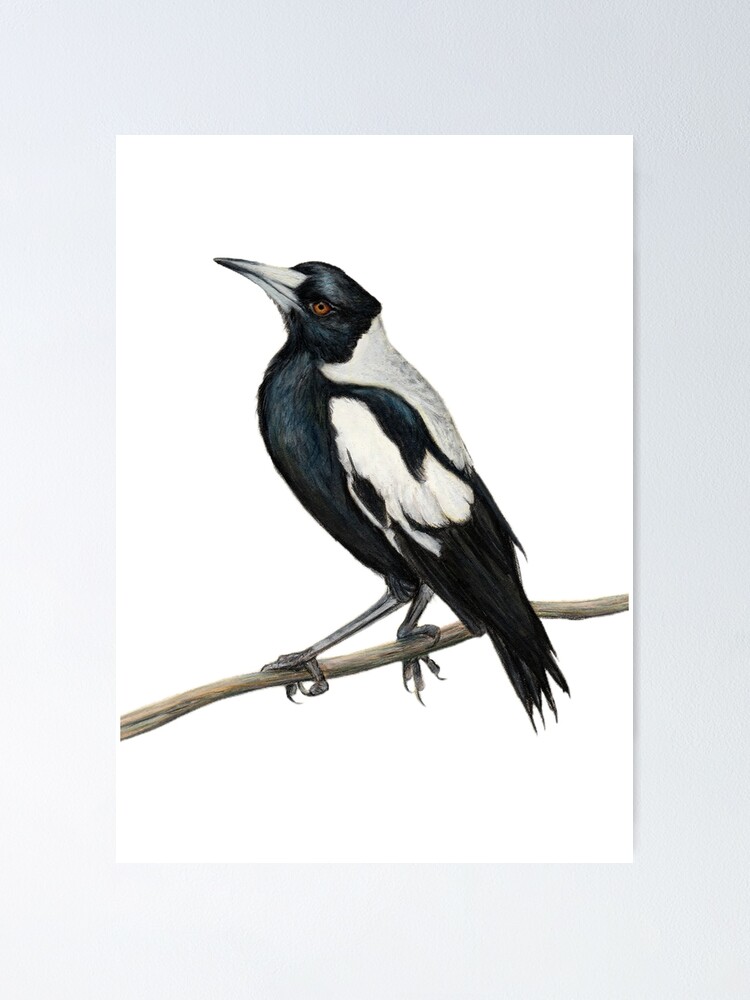The image is a vertically rectangular multi-colored print piece, encased in a thick blue border that fades significantly from the lower left-hand corner to the lower center and along a large part of the left-hand side. Within this border, there is a white, vertically rectangular paper, approximately 8 by 10 inches in size. The central focus of the print is an artistically interpreted bird perched on a slender, brown branch. The bird is oriented towards the left side of the frame, showcasing intricate details: a pointed white beak, and striking red eyes. Its head and chest are black, while its back is mostly white, extending from the nape of the neck down to mid-back. The wings feature a distinctive black and white feather pattern, arranged in a hook design, and the tail is entirely black. The frame surrounding this composition is purplish, and the background within the frame is a plain white, accentuating the bird's vibrant and detailed appearance.